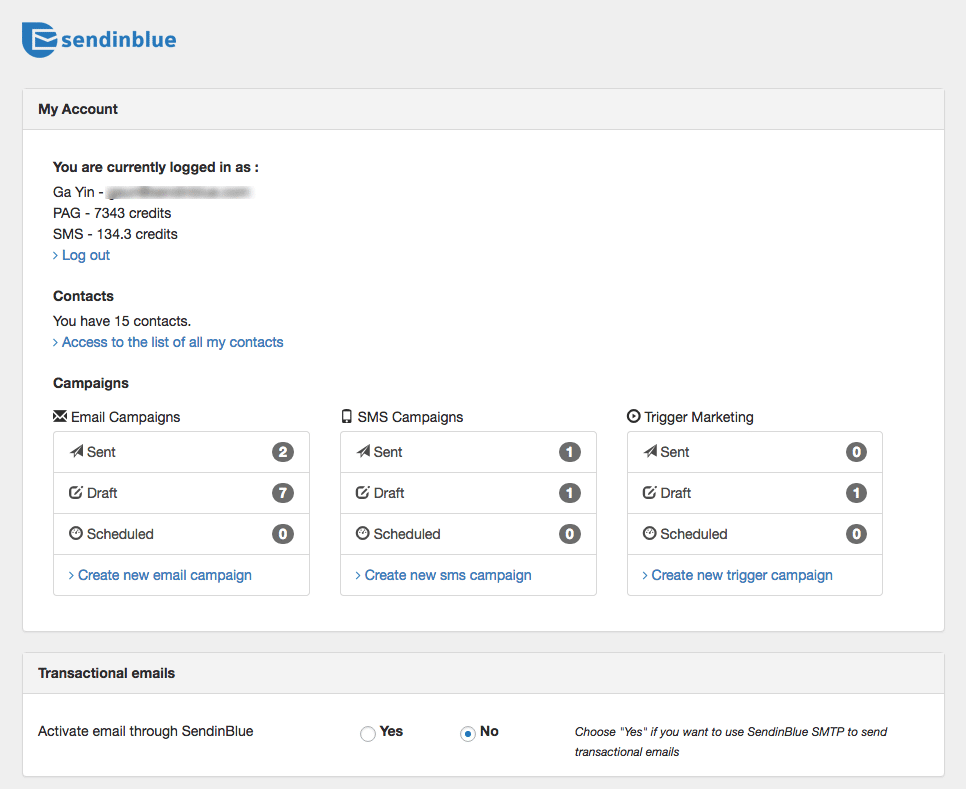A detailed screenshot from an email marketing platform (possibly Sendinblue) is displayed. The interface reveals various account details and functionalities:

- **User Information**: The user is currently logged in as "guy in with blank."
- **Account Details**: The user’s account is associated with 7343 SMS credits and 134.3 email credits. There is an option to log out.
- **Contacts**: The user has 15 contacts, with an option to access the full list.
- **Email Campaigns**:
  - Sent: 2
  - Drafted: 7
  - Scheduled: 0
  - Option to create a new email campaign.
- **SMS Campaigns**:
  - Sent: 1
  - Drafted: 1
  - Scheduled: 0
  - Option to create a new SMS campaign.
- **Trigger Marketing**:
  - Sent: 0
  - Drafted: 1
  - Scheduled: 0
- **Transactional Emails**: 
  - Activation Option: There is a toggle to activate email sending through Sendinblue SMTP. Currently, the "No" option is selected. A note indicates that users can choose "Yes" if they want to send transactional emails through Sendinblue SMTP.

The user comments on the functionality, remarking that it appears to be a system designed to send mass emails, possibly implying it could be used for spam.